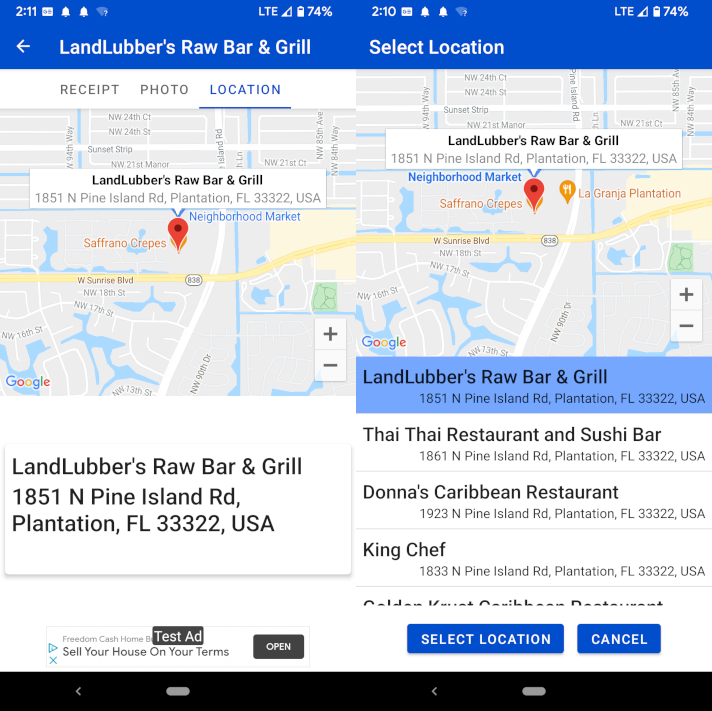**Detailed Caption for the Image:**

The page displays two screenshots from an iPhone. The first screenshot shows the top status bar with the time displayed as 2:11 PM and the battery level at 74%. Just below the status bar, there's a blue navigation bar indicating the name "Landlubber Raw Bar and Grill." 

The main part of the screen features a map highlighting the location of this restaurant. The address is specified as 1851 N Pine Island Road, Plantation, Florida 33322, USA. A location icon pinpoints the exact spot of the restaurant. The map also includes various elements: a prominent yellow line representing a curved roadway, white lines defining other roads and streets, and blue, curvy lines illustrating nearby water bodies.

Right below the map, there is a promotional text ad urging users to "sell your house on your terms," accompanied by an "open" button on the right. Further down, the text "Landlubber Raw Bar and Grill" is listed again, followed by other local establishments such as "Thai Thai Restaurant and Sushi Bar," "Donna's Caribbean Restaurant," and "King Chef."